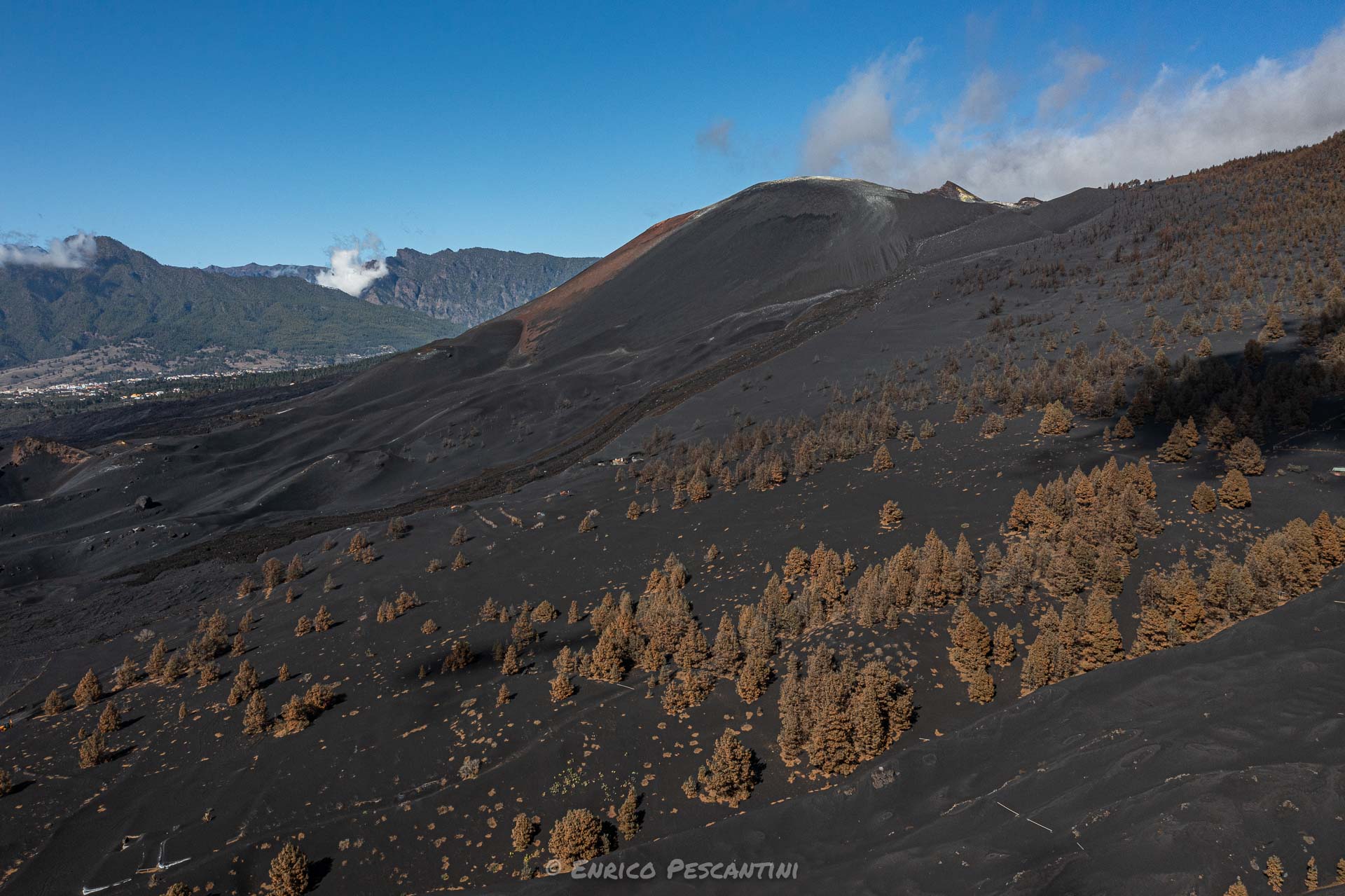The photograph depicts an aerial view of a stark, barren mountainside, seemingly ravaged by a wildfire or volcanic activity. The slope is coated in a dark, almost charcoal-like ash, punctuated by sparse conifer trees that appear dry and lifeless, their hues ranging from yellowish-beige to deep brown. Some areas of the mountain are nearly blackened, emphasizing the extent of the damage. In contrast, the distant background features verdant, green mountains shrouded in blue sky and interspersed with white clouds, mist, or smoke. The scene is shot during daytime, as indicated by the clarity of the clouds and the overall brightness. At the bottom center of the photograph, the name "Enrico Tescantini" or "Enrico Pasquantini" is visible, presumably attributing the image to the photographer.